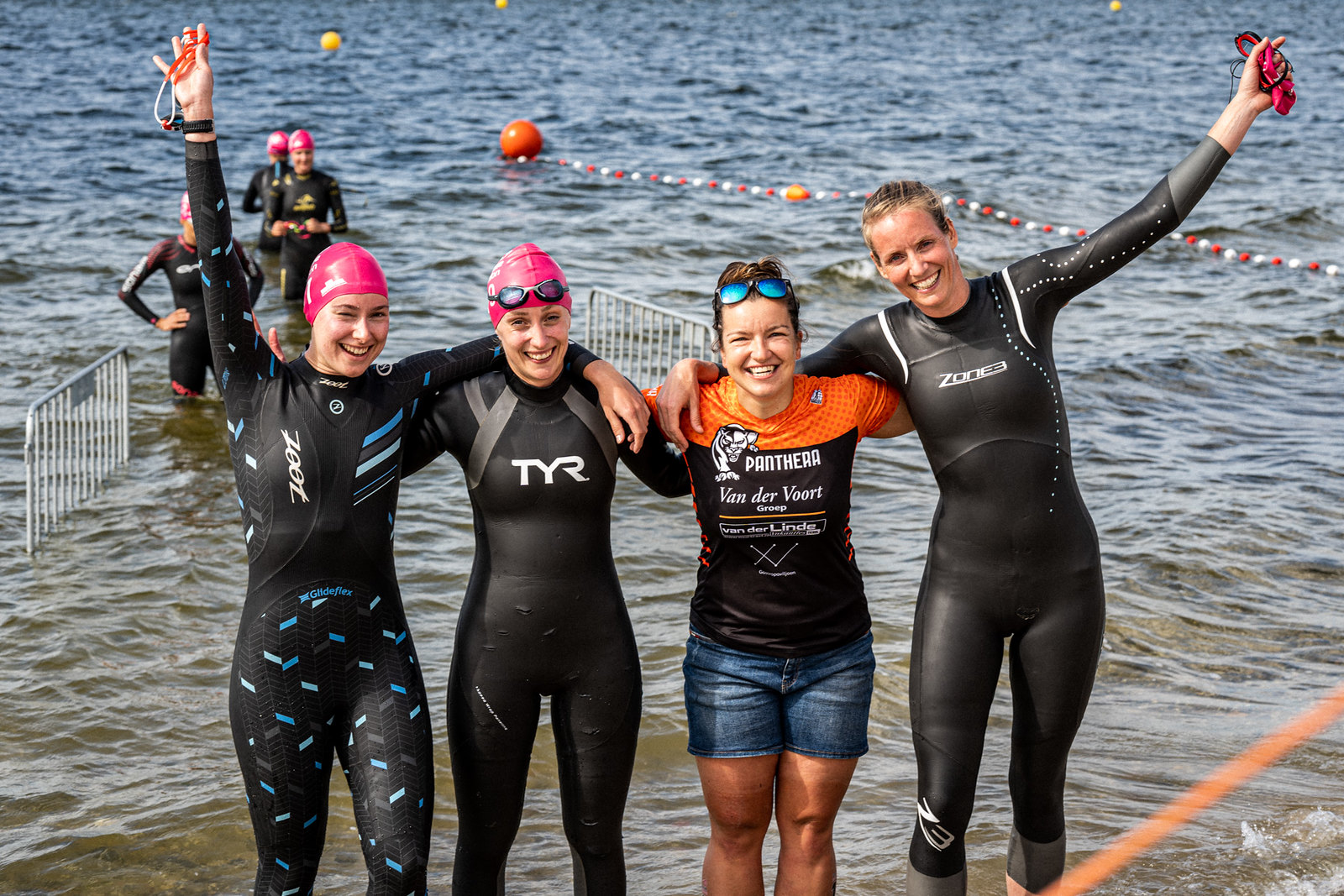Four women, all dressed in sleek black full-body swimsuits, pink swim caps, and goggles, stand smiling triumphantly in a river. They have just completed an underwater swimming event, marked by their raised hands and joyous expressions. The sunny weather highlights their happiness and the celebratory atmosphere around them. Behind the women, three individuals, one of whom is conspicuously dressed in a shirt with yellow accents rather than swim gear, stand observing the scene. Buoys dot the water, adding context to the racing event.